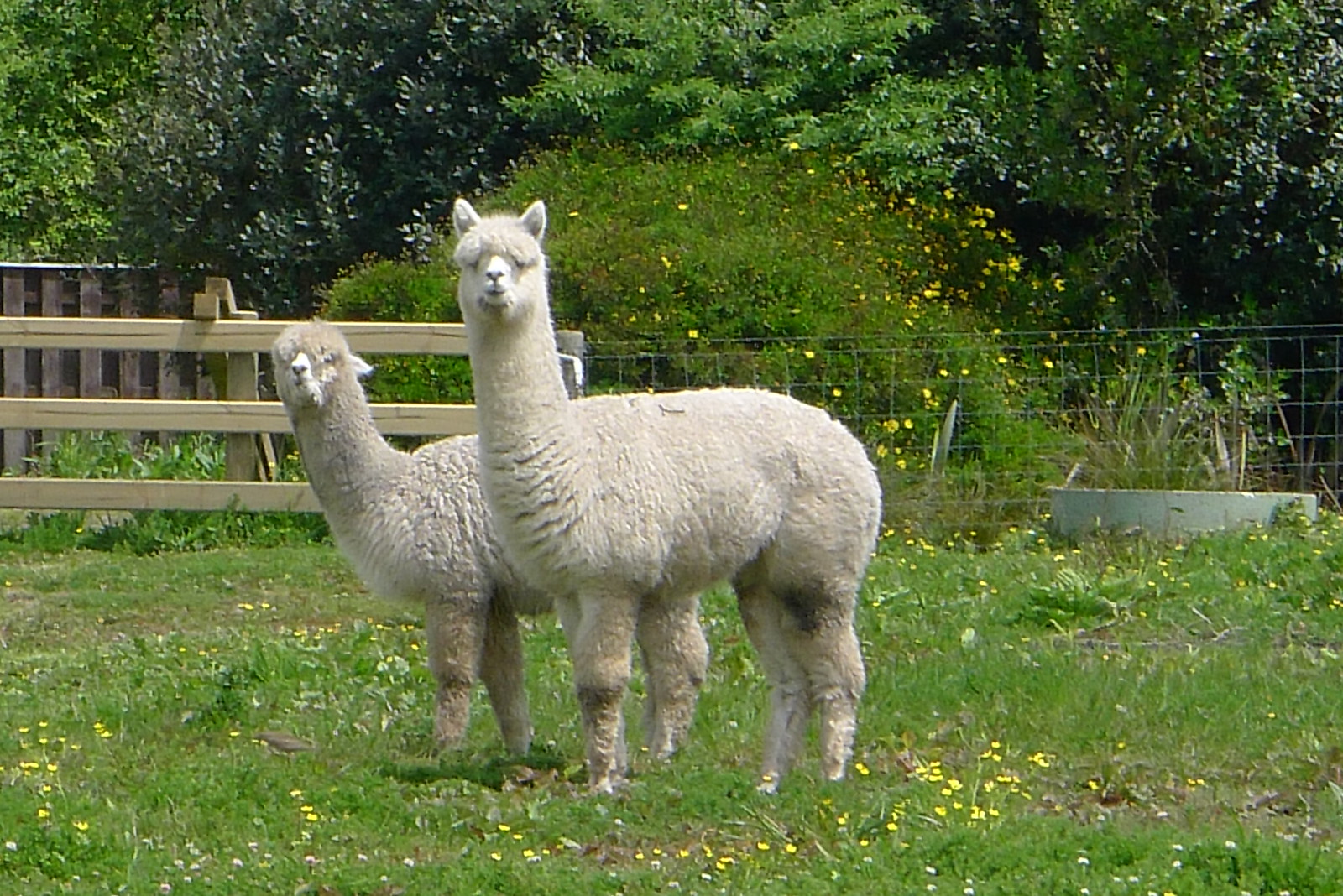In a lush, green field dotted with vibrant yellow flowers, two llamas stand attentively, both gazing directly into the camera. One llama, slightly smaller and white in color, has its ears down, portraying a more subdued stance. The other, taller and equally white llama, has its ears perked up, exuding a curious demeanor. Behind them, a wooden fence with three horizontal cross beams and a vertical post is visible, alongside a wire fence. The background features a low concrete wall forming the base of more wire fencing, which extends into a dense grove of trees interspersed with the same yellow flowers found in the field. The scene captures a serene outdoor setting, free from any people, buildings, or vehicles, emphasizing the natural beauty and surroundings of the llamas.